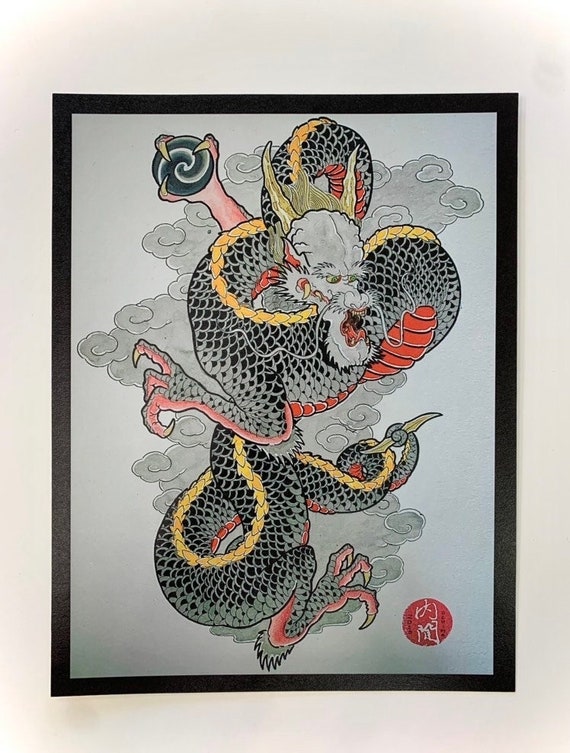This is a color photograph of a traditional Japanese-inspired poster displayed on a white wall. The image features an Asian dragon set against a cream tan colored background, framed by a sleek black rectangular border. The dragon possesses a fierce, demon-like face with white scales, embellished with long whiskers, a prominent beard, and large golden horns. A striking golden stripe runs along its predominantly black-scaled body, tinged with gray. The dragon’s underbelly and some of its feet are highlighted with red scales. Its formidable claws and talons are tinged with a pinkish-red hue. The dragon’s sinuous body coils snake-like around the composition, ending in a tail that curls around a small golden item. Outstretched, its arms display menacing claws, one of which precariously holds an enigmatic, glass or jade-colored orb. This orb, dark gray in color with a swirling, tornado-like design, evokes a sense of magical potency. In the background, wisps of gray clouds add depth and mystique to the scene. The artist’s signature, written in Japanese characters, sits subtly within the illustration, reinforcing its traditional aesthetic.